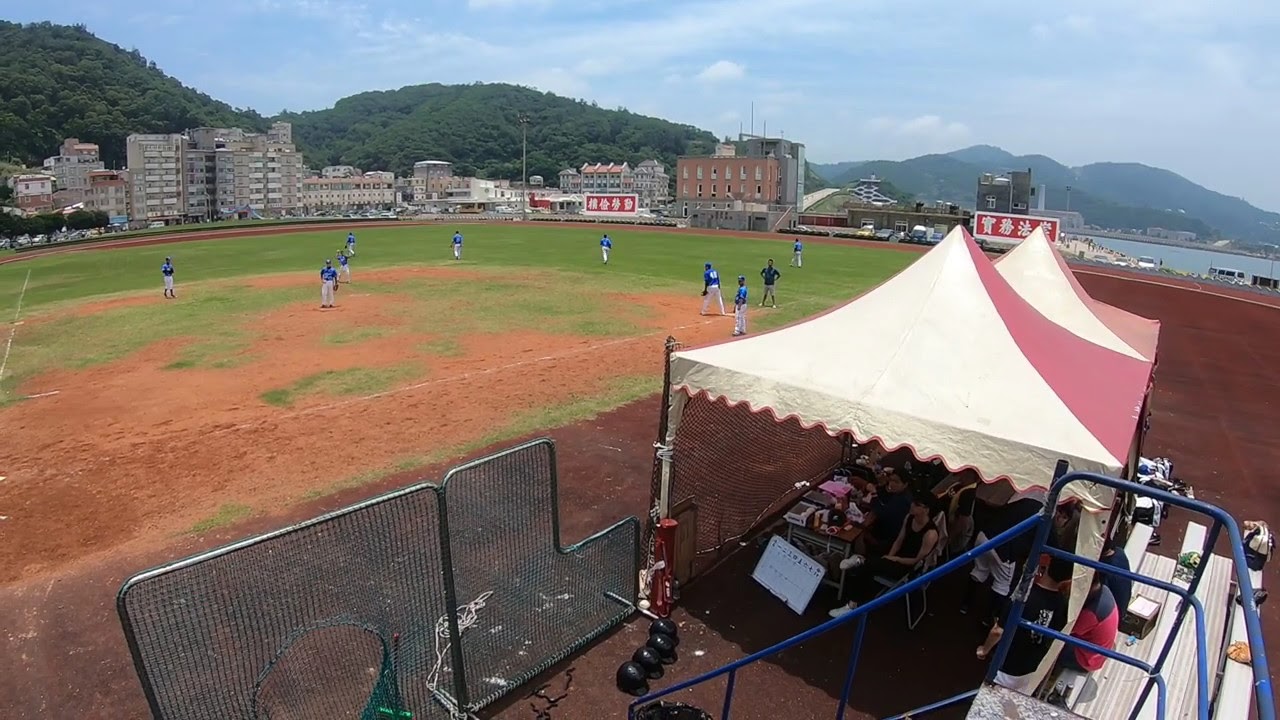This high-resolution photograph captures an overhead view of a baseball game in progress. The field is a well-worn mix of green patches interspersed with large areas of brown dirt, indicative of frequent play. The players, dressed in blue jerseys and gray pants, appear small from this vantage point, suggesting the photo was taken from high up in the stands, where blue rails are visible in the lower right corner. On the perimeter of the field, two red and white tents house spectators seated in chairs, adding to the bustling atmosphere. The background reveals a picturesque landscape of tall green hills dotted with trees, a body of water, and an urban scene of multi-story brown and beige buildings, suggesting a location possibly in China, as indicated by red signs with Chinese characters. The sky above is a soft blend of blue with hazy clouds, enhancing the bright and clear daytime setting.